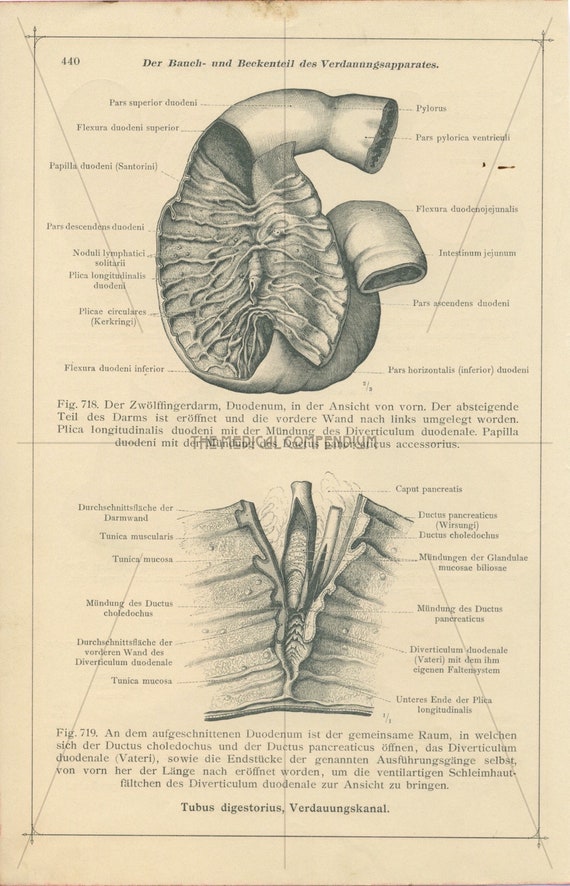The image is a detailed pencil diagram on a faded beige, parchment-like page, seemingly extracted from an old encyclopedia or a medical book, specifically page 440. The content is primarily in German, suggesting an international origin. The top section of the page is bordered by black lines and features a central organ, which is likely a detailed depiction of the human stomach, showcasing its internal structure with numerous valleys and connecting tubes at both ends. Surrounding the organ illustration are extensive labels in German, pointing to various anatomical parts, with terms like "Pelorus" and "Parse Pelorus Ventricle" identified. Beneath this is another smaller diagram, probably illustrating different anatomical features, potentially layers of the skin including the epidermis, dermis, and fascia, all accompanied by explanatory text. The text also contains a paragraph describing the figure, marked as figure 719.